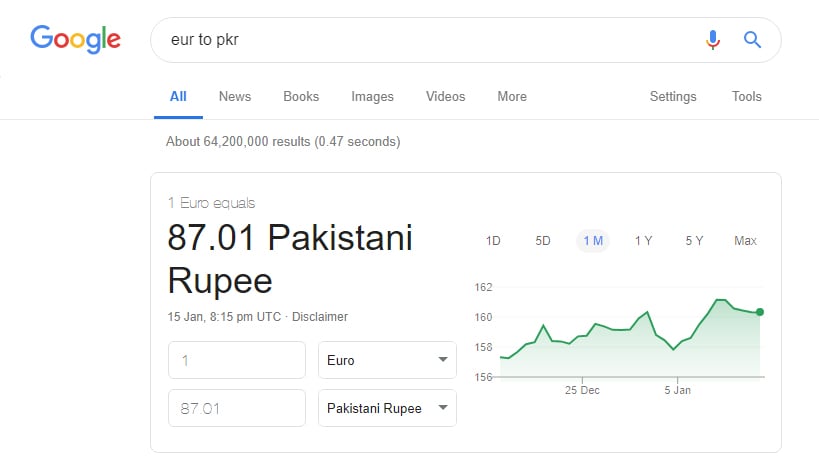This desktop screenshot from a Google search illustrates the results page for the query "EUR to PKR" (Euros to Pakistani Rupees conversion). At the top of the page, the current exchange rate is prominently displayed, showing that 1 Euro equals 87.1 Pakistani Rupees as of January 15th at 8:15 PM UTC, with a disclaimer noting the timestamp and possible variations.

Below the main conversion rate, there are input fields allowing users to convert different amounts of Euros to Pakistani Rupees and vice versa. The default setting shows the conversion for one Euro, which equals 87.01 PKR. 

On the right side of the conversion result, a small line graph presents historical exchange rate trends over the past month, marked as "1M." This graph visually depicts the fluctuations in the exchange rate, highlighting peaks and valleys that signify the highs and lows over this period.